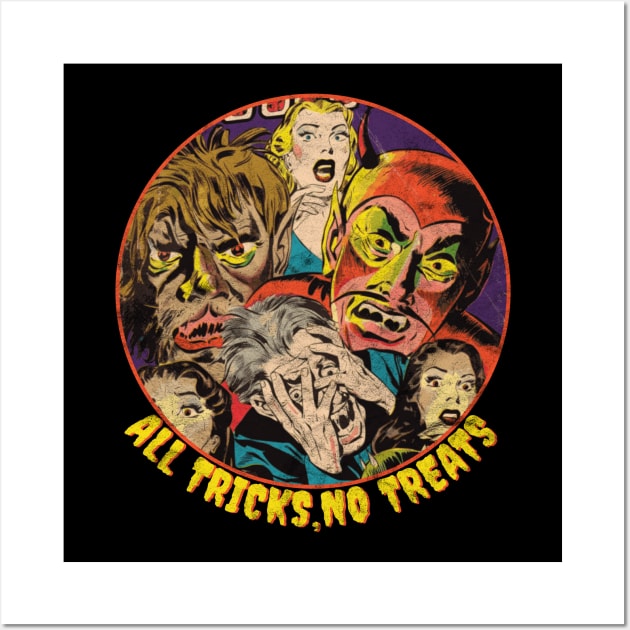This is an illustration with a distinct 1950s style, set against a solid black background. At the center is a red-lined circle containing a haunting scene featuring six cartoonish figures, all of whom appear terrified. The top of the circle shows a blonde woman with red lipstick, screaming in terror. To her left, there's a man transforming into a werewolf, depicted with shaggy brown hair and growing facial fur. On her right, a figure in a devil costume with a thin black mustache, pointy teeth, horns, and pointy ears adds to the macabre scene. Below them, an elderly man with gray hair covers most of his face with his hands, his mouth open in a scream. To his left, partially visible, is a woman with black hair, and to his right, another woman with long brown hair, both of whom appear equally horrified. The image is framed by a white mat, and beneath this chilling tableau, a yellow caption reads, "All tricks, no treats."